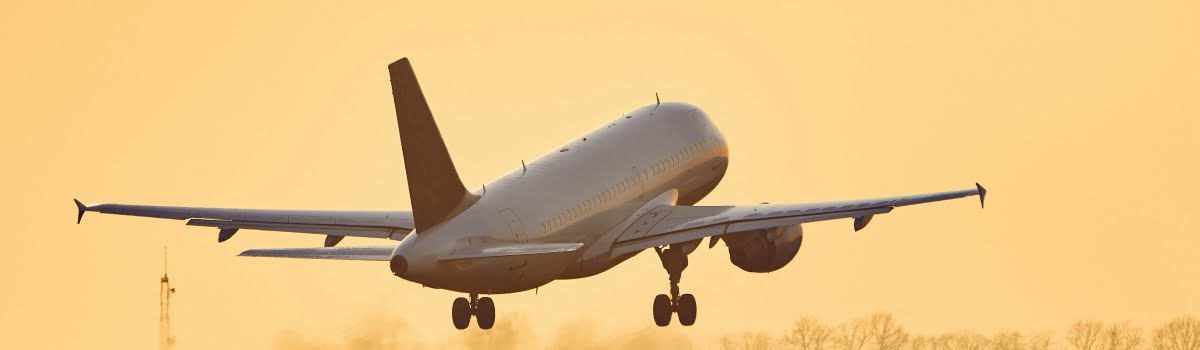This color photograph captures a medium-sized airplane, likely a Boeing 737 or similar, taking off into a sky shrouded in a thick, orange-tinted haze. The airplane, predominantly white with a dark-colored tail, is photographed from behind, and its landing gear is still extended, indicating it has just lifted off. The sky's unnatural glow suggests the presence of a heavy dust storm or severe pollution, obscuring the landscape and casting a surreal, almost apocalyptic filter over the scene. Along the bottom of the image, faint silhouettes of trees and metal structures, including what appears to be a radio tower, are barely visible through the murky air. The plane's wingtips feature small, triangular extensions, adding a unique detail to its profile as it climbs away from the obscured horizon.